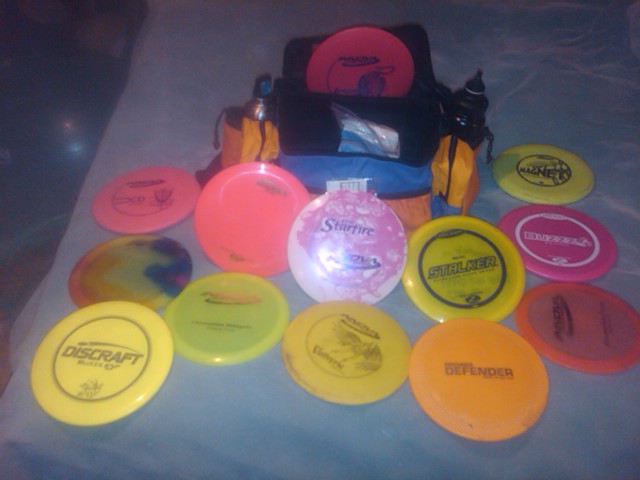This slightly out-of-focus photograph depicts a collection of twelve disc golf discs laid out on a light surface, possibly a white rug or sheet, with intricate and colorful designs. Among the discs, which vary in colors such as yellow, pink, orange, and a multicolored tie-dye pattern, several brand names and models can be identified: Discraft, Defender, Stalker, Starfire, and Magnet. The shot appears dim, suggesting it might have been taken at night in a bedroom setting, partially revealing a wooden floor and a large balance yoga ball in the background. Centrally positioned is a canvas duffel bag, predominantly yellow and blue with black accents. It features dual water bottle holders—one containing a silver bottle and the other a black one. From the bag's main compartment, a pinkish-blue disc is visible. The image has a flash-induced shine, which adds to the overall blur and uneven focus.